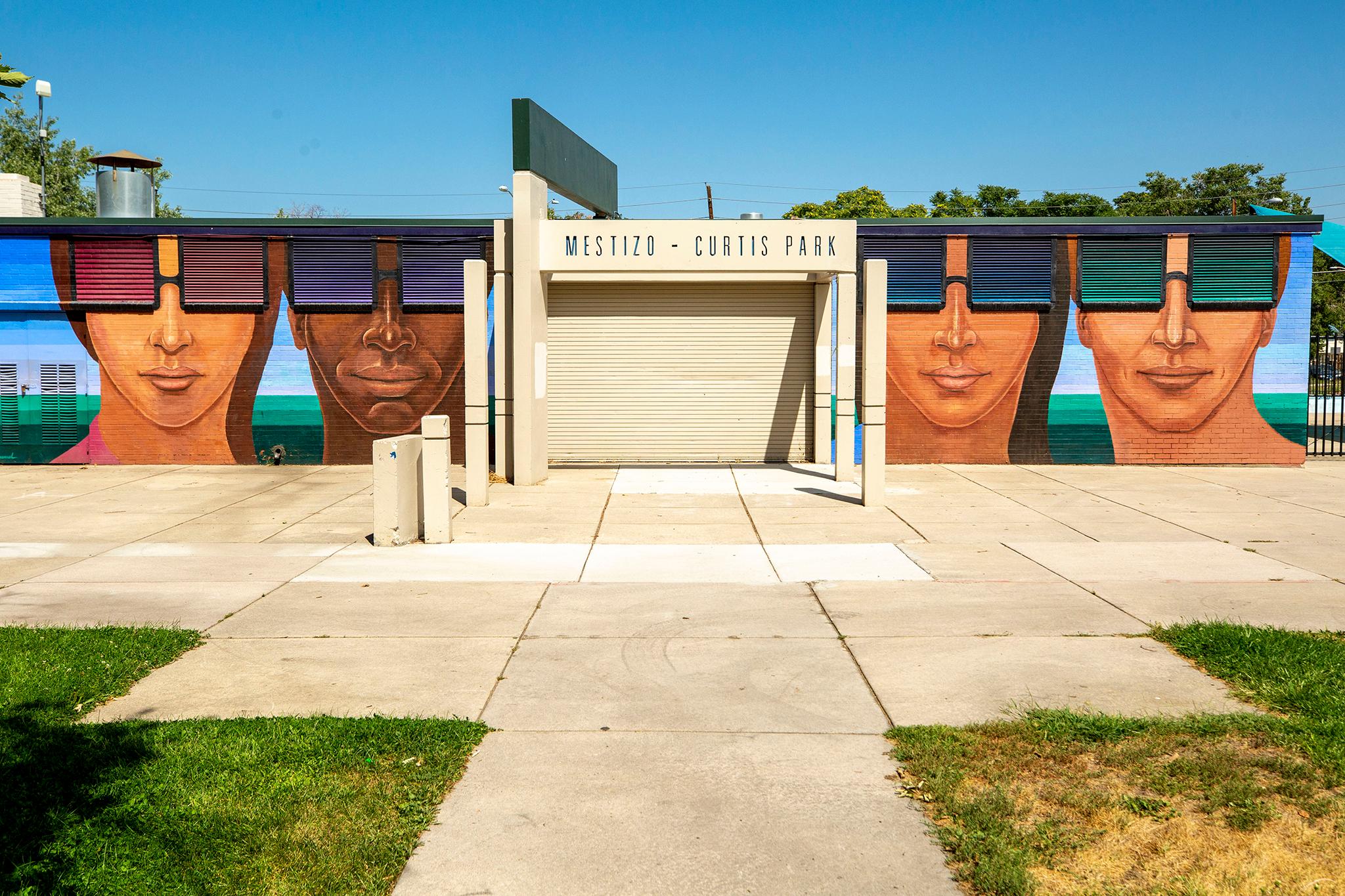The photograph captures the side of a modern one-story building adorned with a striking mural at Mestizo-Curtis Park. The mural features four large human faces, two on each side of a central garage door. These faces are distinctive because the building's window blinds are cleverly incorporated as large square sunglasses, adding a unique artistic touch. 

On the left side of the doorway, a white woman and a black man are depicted, each appearing to wear these innovative sunglasses. On the right, a long-haired individual and another white person are portrayed in a similar fashion. 

The foreground consists of a beige and white cement pathway leading to a spacious courtyard with large pavers. There is grass on the left, and some dead grass to the right, framed by a cast iron fence. The sky is a cloudless, vivid blue, and trees rise behind the building, completing this sunlit, urban artwork scene.